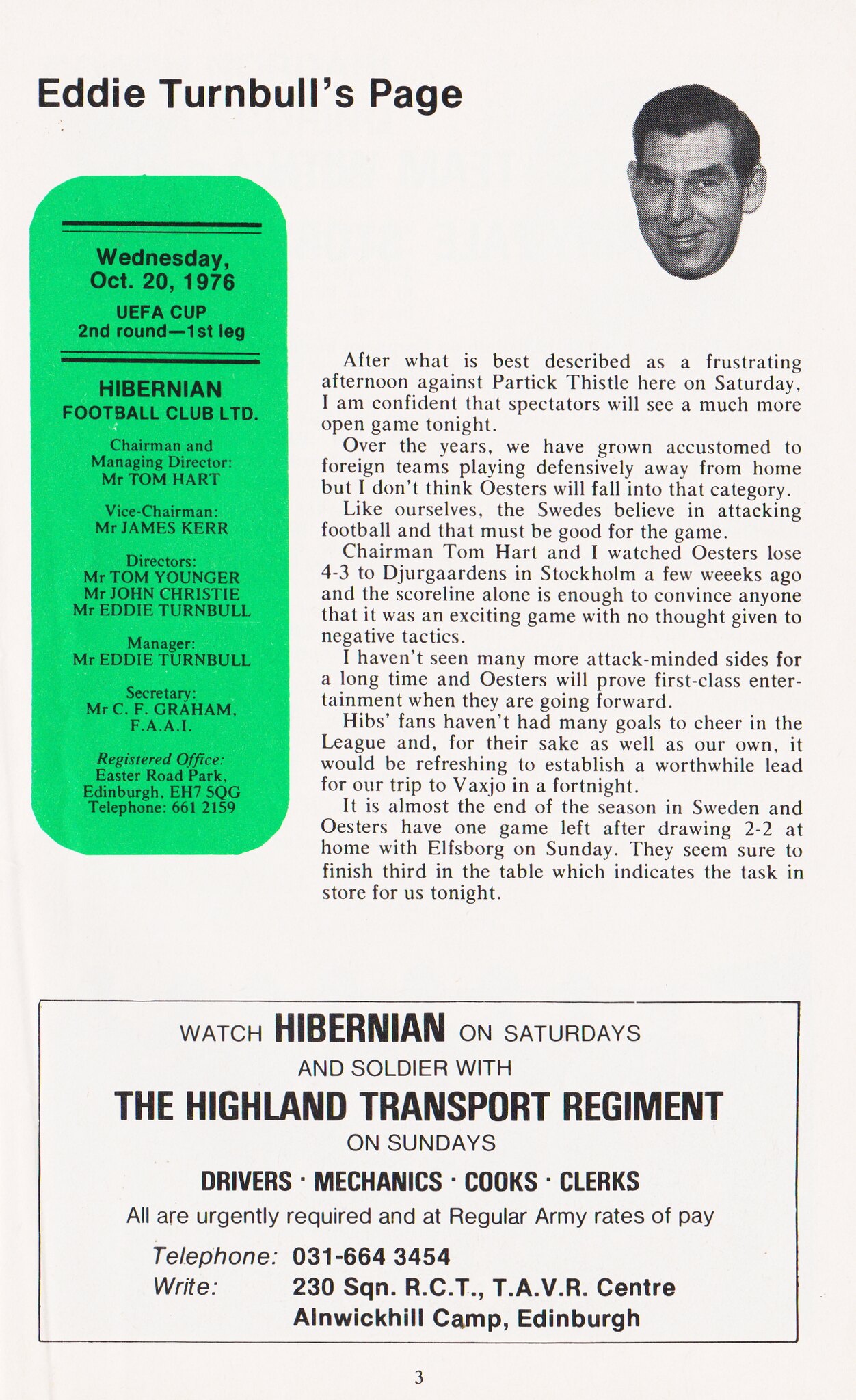The image depicts a magazine or newspaper article page titled "Eddie Turnbull's Page" in the upper left corner. In the upper right corner, there's a black-and-white headshot of an older white man with dark hair and thick eyebrows. Below the title, and starting on the left side of the page within a long green rectangle, is detailed information dated Wednesday, October 20th, 1976, about the UEFA Cup second round, first leg. It lists the Hibernian Football Club Limited's key personnel: Chair and Managing Director Mr. Tom Hart, Vice Chairman Mr. James Kerr, Directors Mr. Tom Younger, Mr. John Christie, Mr. Eddie Turnbull, Manager Mr. Eddie Turnbull, and Secretary Mr. C.F. Graham, FAAI. The registered office is located at Easter Road Park, Edinburgh, EH7 5QG, alongside a telephone number.

The main body of the page, set in black text on a white background, appears to contain a lengthy biography or article. At the bottom of the page, within a small white square, there's an advertisement encouraging people to watch Hibernian on Saturdays and join the Highland Transport Regiment on Sundays. It highlights the need for drivers, mechanics, cooks, and clerks at regular Army rates of pay, followed by contact information.